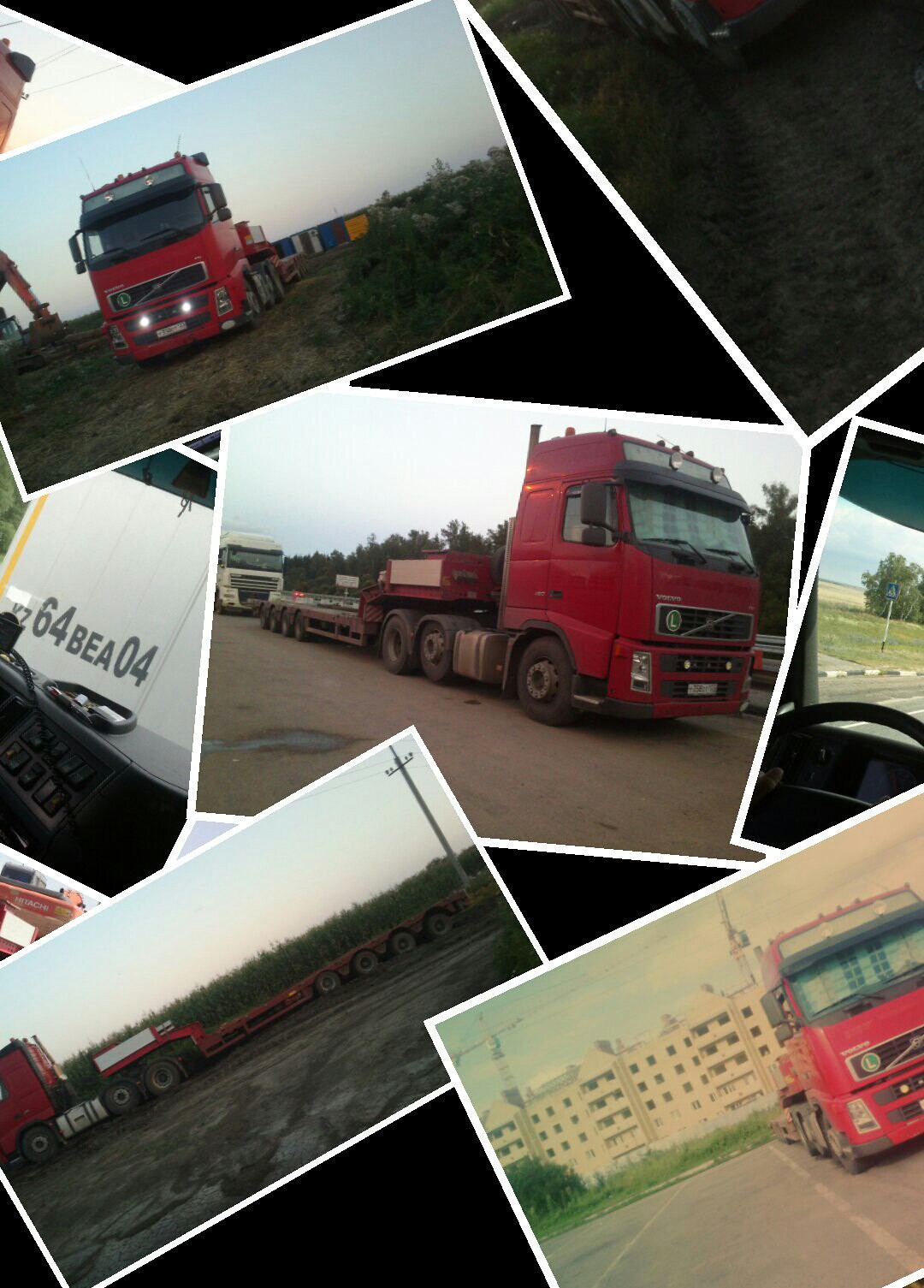The image is a vintage-style collage postcard, likely from the early 90s, featuring a series of photographs of a red flatbed truck. The collage includes about four or five pictures of the truck, each taken from different angles and settings. One image shows the truck against a blue sky with no trailer attached, while another captures it driving down a city street with tall buildings in the background. Other pictures show the truck on flat fields, dirt roads, and accompanied by telephone poles. The photographs are arranged unevenly with some diagonally and the central image slightly tilted, each bordered in white. The dark wooden table beneath the postcard adds a contrasting backdrop. Notably, one image includes text marked as "K764BEA04," potentially identifying the truck's model.